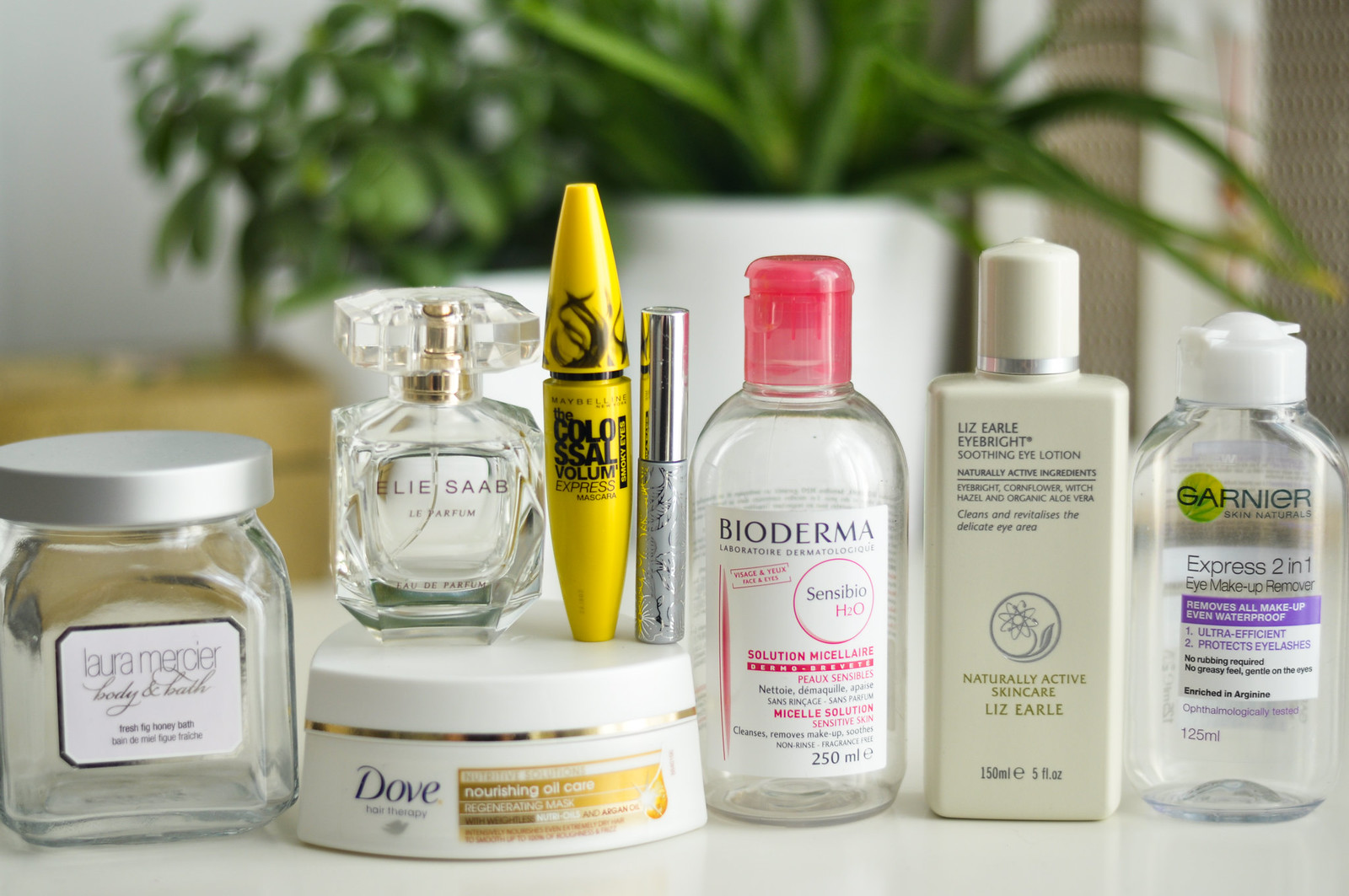This image captures a pristine white countertop adorned with an array of beauty products, each meticulously placed in line. On the far left, there's an elegant glass jar with a silver screw-top lid. The label displays "Laura Mercier Body and Bath" with "Fresh Fig Honey Bath" elegantly scripted across a white background with gold trim, though the jar is currently empty.

Next in line is a unique, softly triangular, white container marked "Dove Nourishing Oil Care." The label features gold accents with "Dove" in signature blue, and "Hair Therapy" noted beneath.

Placed atop the Dove container is a sophisticated glass perfume bottle complete with a glass lid, brandishing the name "Elie Saab Le Parfum" in fine print across its surface.

Directly atop the Dove Hair Therapy is a vibrant yellow tube of mascara. The striking packaging reads "The Colossal Volume Express, Maybelline."

Adjacent to it stands another mascara tube, this time silver with a matching silver top, adorned with delicate silver floral designs towards the bottom of the tube.

Further along the countertop, there's a clear plastic bottle of face care product labeled "Bioderma." It features a pop-top lid in a cheerful pink hue.

Following this is a tan bottle with a coordinating tan screw-top lid lined with silver. It reads "Liz Earl Eye Bright Soothing Eye Lotion," with a fanciful "Earle" spelling.

Finally, there is a plastic bottle containing Garnier Skin Naturals Express 2-in-1 Eye Makeup Remover. The bottle is capped with a white pop-top lid, completing the diverse collection of skincare and beauty products gracing the countertop.